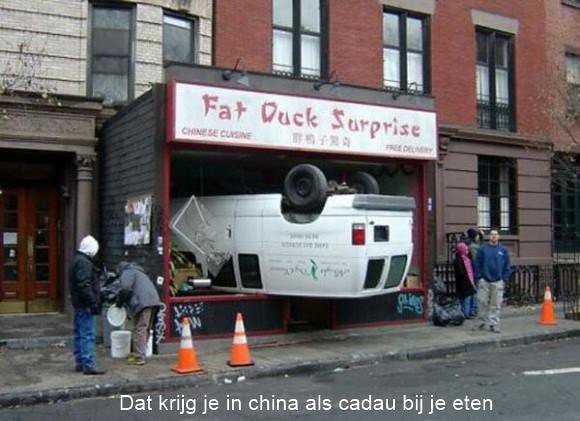This photograph, likely taken in the early days of digital photography judging by its quality, captures a dramatic scene outside a building with residential units above and a commercial area at its base. Centered prominently is a white van that has crashed and flipped upside down into a Chinese restaurant named "Fat Duck Surprise." The restaurant's signage features the text "Chinese cuisine," "free delivery," and some Chinese characters, all in red on a white background. The exterior of the restaurant is predominantly black with red accents outlining its edges and corners, creating a visually striking contrast. The building itself is part of a larger structure with a mix of grey, red, and brown colors, and features a door to its immediate left. The shop juts into the sidewalk, which is angled lower on the left and higher on the upper right side of the photo. Multiple people are seen milling about on either side of the restaurant, adding to the chaotic atmosphere. Three orange traffic cones are placed along the sidewalk, two directly in front of the shop and one further to the right. The surrounding buildings include a red brick one on the right and a white brick one on the left. Notably, text in a language that appears to be Swedish or Norwegian is visible at the bottom of the photo, emphasizing the scene's international intrigue.